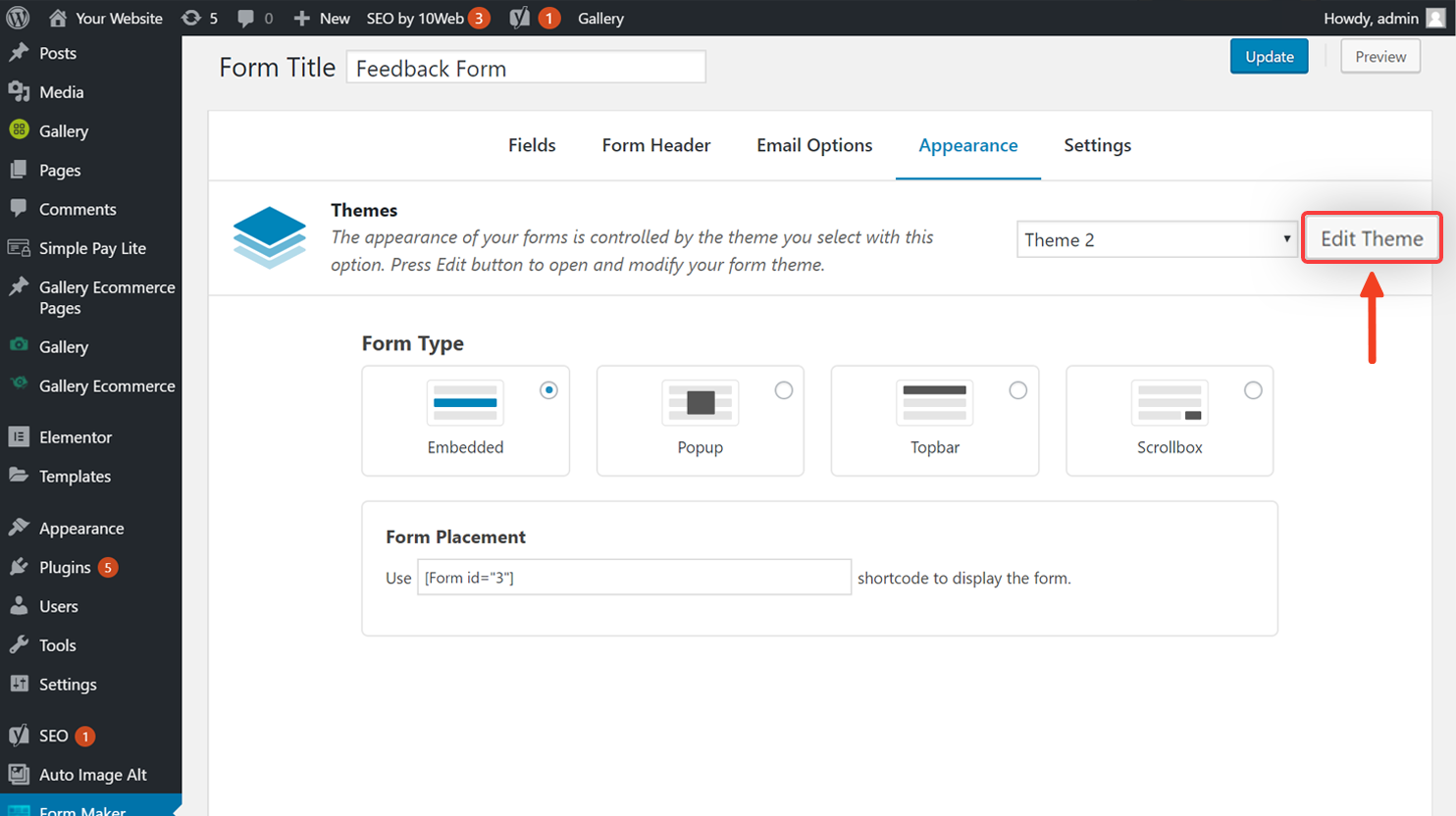The screenshot depicts the interface of a WordPress dashboard. The navigation bar on the left-hand side features a comprehensive list of menu items, including "Posts," "Media," "Gallery," "Pages," "Comments," "Simple Pay," "Gallery" (repeated three times), "E-commerce," "Elementor," "Templates," "Parent," "Plugins," "Users," "Tools," "Settings," "SEO," and "Auto Image."

On the right-hand side of the dashboard, the section is titled "Form Title," followed by configuration options such as "Field," "Form," "Email Options," "Appearance," and "Settings." A prominent red box highlights the "Edit" function under these options. 

Further down, there is a section labeled "Theme" with a dropdown indicated as "Theme 2," allowing the user to select from five different form display options: "Embedded," "Pop-up," "Top Bar," "Scroll," and "Form Placement." Additionally, it mentions the use of a shortcode to display the form.

A red arrow points upward towards the "Edit Theme" option. At the bottom of the interface, there's a reference to "SEO by 10Web," accompanied by a circular icon containing the number three and another solid circle with a number one inside it.